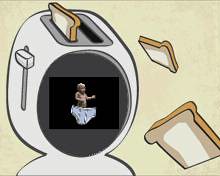The illustration is a computer-generated drawing with a beige background, showcasing an abstract and whimsical depiction. On the left side of the image, there is a quirky character resembling a cross between a spaceman and an Eskimo, with a head shaped like a white toaster. The top of this toaster-head is flat, featuring two grey slots, one of which has a piece of toast popping out. Where the character’s ear would be, there's a slider lever, similar to those found on traditional toasters. 

The toaster character displays a detailed front, incorporating a dark grey panel with a black square screen. Within this screen, a small child with blonde hair is depicted, dressed in an oversized pair of whitish Y-front underpants that appear as an exaggerated diaper. The child’s lower body is entirely encased in these enormous underpants, contributing to the surreal aspect of the illustration. 

Additionally, the background includes two pieces of toast floating on the right-hand side, appearing as though they are suspended in mid-air. The image stylistically presents the toaster and baby elements in a unique and imaginative manner, blending everyday objects with an unusual artistic twist.